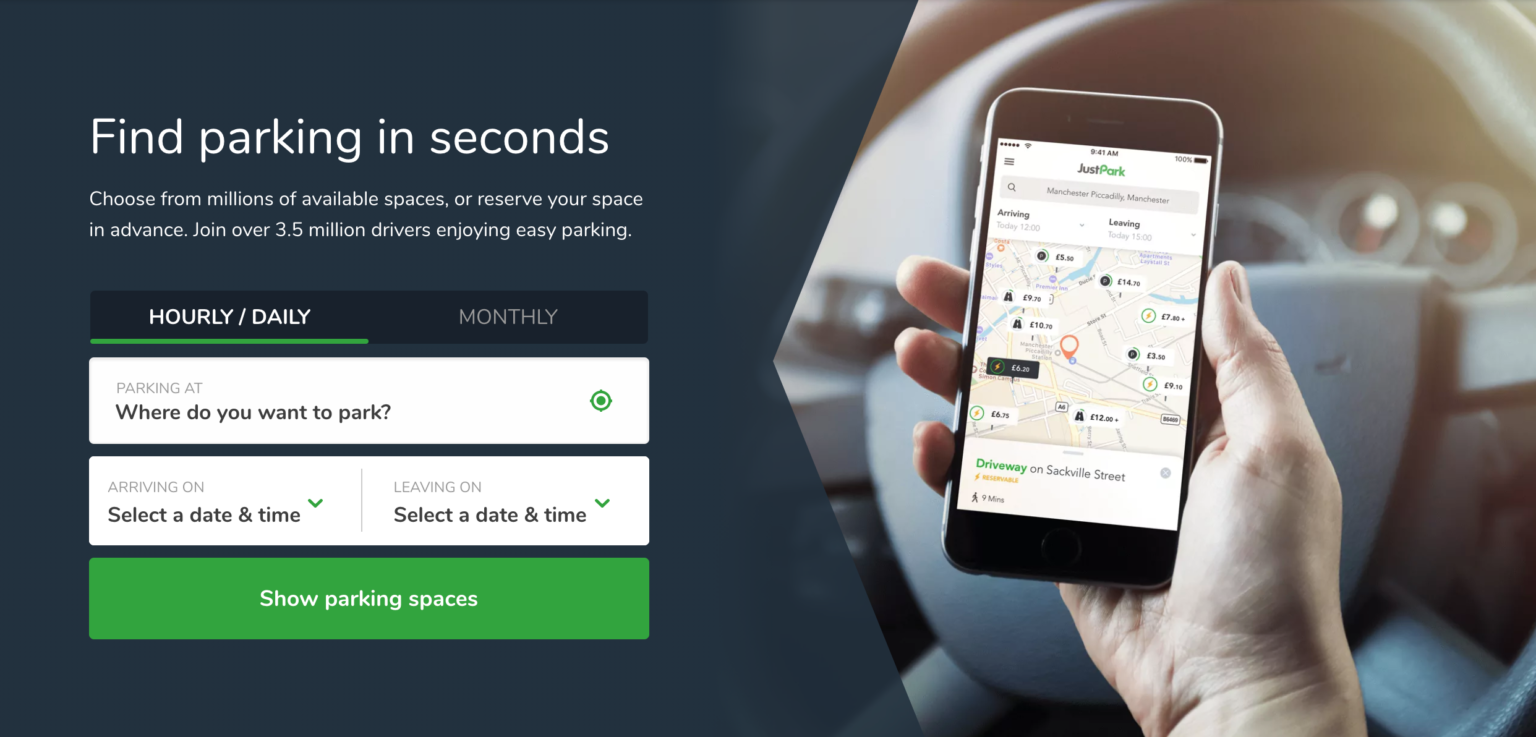This is a detailed description of an image depicting a web page or app interface for finding parking spaces. The image is horizontal and divided into two distinct sections. 

On the left side, the background is a navy blue color with the following text in white:
- The main heading says "Find parking in seconds."
- Below the heading, in a smaller font, it reads, "Choose from millions of available spaces or reserve your space in advance. Join over 3.5 million drivers enjoying easy parking."
- A black strip follows with "Hourly / Daily" in white and "Monthly" in gray. A green underline emphasizes "Hourly / Daily."
 
Further down, a white rectangular box contains the text "Parking at" followed by the prompt "Where do you want to park" in black. To the right of this box is a green button.

Another white rectangular box below says "Arriving on" with the option to "Select a date and time" indicated by an arrow pointing down. A gray line separates this section from another that reads "Leaving on," followed by the same "Select a date and time" prompt in black.

At the bottom, a green rectangular button with white text reads "Show parking spaces."

On the right side of the image, a partial view of a car's interior is shown. The dashboard and steering wheel are visible, along with a Caucasian hand holding a smartphone. The phone's screen displays the "JustPark" app, suggesting that the person is in the process of finding or reserving a parking space using the app.

Together, the image portrays the functionality and user interface of a parking application designed to simplify finding and reserving parking spots.